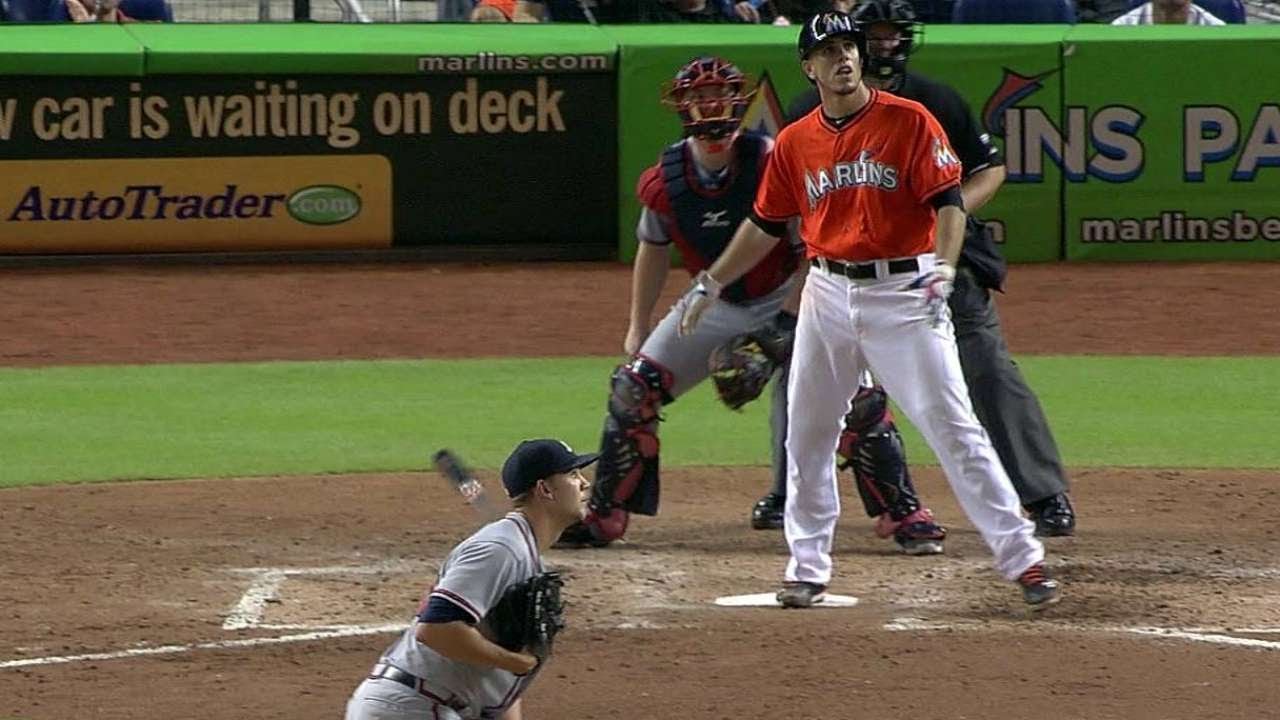This image captures a moment during a Major League Baseball game, likely featuring the Miami Marlins at their home field, given the visible "Marlins.com" advertisements and partially obscured Marlins logo on the outfield fence. The scene shows four central figures — the pitcher, the batter, the catcher, and the home plate umpire. The batter, wearing the Marlins' signature orange jersey and white pants, stands on home plate, watching intently towards the right side of the frame, suggesting he has just hit the baseball, possibly a home run given that his bat is already out of his hand.

The pitcher, dressed in a gray uniform with a blue cap, mirrors this gaze, his focus directed towards the path of the ball. Behind the batter, the catcher, clad in his protective gear including a mask, vest, and shin guards, and the umpire, distinguishable by his black shirt and gray pants, both look towards the same direction, confirming the trajectory of the hit. The presence of the audience at the top of the photo adds to the atmosphere, with their attention fixed on the action unfolding on the field. The layered advertisements, including one for "autotrader.com" with a truncated slogan, frame the upper perimeter of the scene, situating this dynamic moment within the well-defined bounds of a professional baseball stadium.